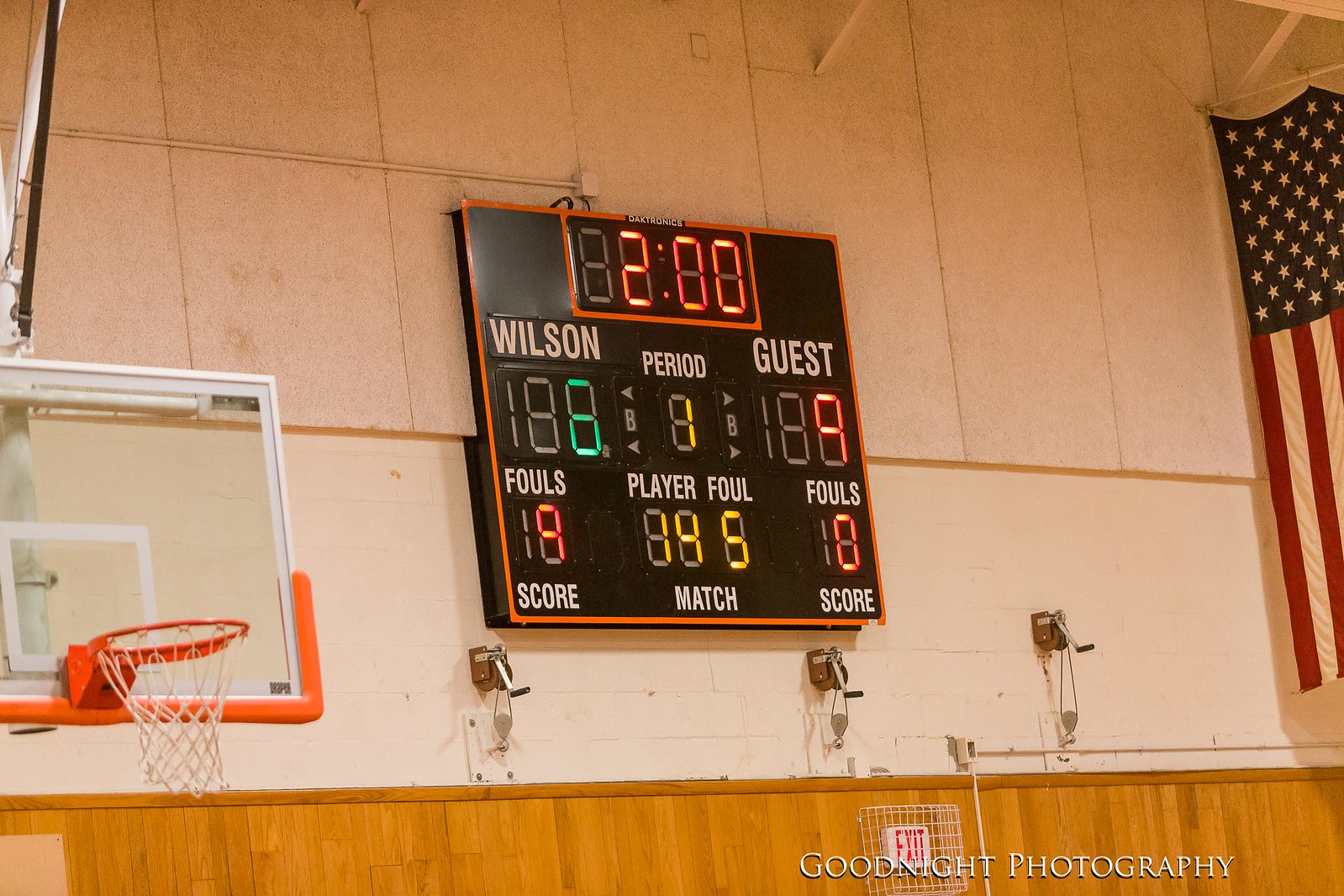This detailed photograph captured by Good Night Photography depicts a high school or university gymnasium, emphasizing the focal points of a vibrant scoreboard and surrounding elements. The scoreboard, mounted prominently on the wall, features various colored sections displaying critical game details: the remaining time is shown as two minutes in orange, Wilson, the home team, holds 6 points indicated by green numbers, while the guests lead with 9 points in red. The period is listed as one, highlighted in yellow. The home team has committed a total of nine fouls, with player number 14 responsible for five of these, all marked in yellow, as compared to the guests who have zero fouls. Adjacent to the scoreboard, a large United States flag is visible in the top right corner, adding to the patriotic decor of the auditorium. On the left side of the frame, an orange basketball hoop with a white net stands out against the gym’s surroundings. Additionally, the bottom right corner of the image is discreetly marked with the label "Good Night Photography" in white text, indicating its credit. The overall capture provides an immersive glimpse into the environment, from game status to cultural elements, within a quaint yet spirited gym setting.